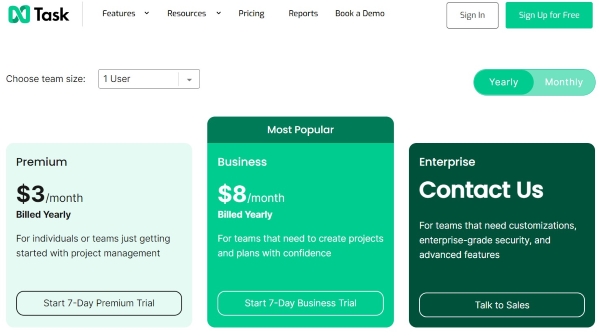The home page of the "Task" application is depicted in this image. At the top left, there is a distinct logo resembling a square-shaped infinity symbol in green, featuring two smaller dark green sections within it. Next to the logo, the word "Task" is displayed in bold, black font. Following a small space and a thin green line, the navigation menu begins, which includes options such as "Features" with a drop-down arrow, "Resources" with a drop-down arrow, "Pricing," "Reports," and "Book a Demo."

To the far right, there are two buttons: a white "Sign In" button and a green "Sign Up for Free" button. Below this menu, on the left side, there's a section to "Choose Team Size," with a dropdown box currently set to "one user." On the right side, there's an oval toggle button split into two segments labeled "Yearly" in darker green and "Monthly" in lighter green.

Beneath these features are three pricing plans displayed in a structured format:

1. **Premium**: Priced at $3 per month, billed yearly. It includes a brief description of benefits, and a button labeled "Start 7-day Premium Trial."
   
2. **Most Popular: Business**: Priced at $8 per month. This plan is highlighted and described as the most popular option, with additional details of the services provided.

3. **Enterprise**: This plan invites potential clients to "Contact Us" for custom pricing and services. It includes a brief description and a button labeled "Talk to Sales."

The image provides an organized and visually appealing representation of the available options and features on the Task application home page.